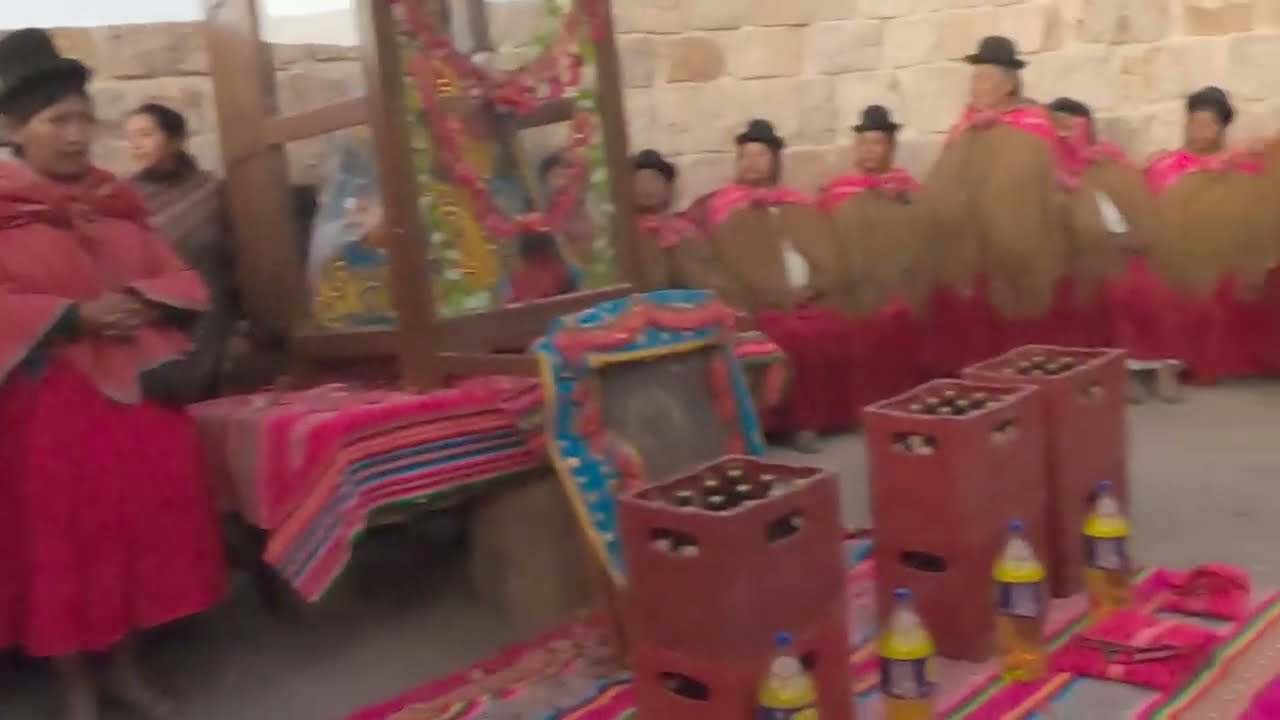In this image, we see a group of six people arranged in a row against a wall that extends beyond the top of the frame, making it hard to determine if the scene is indoors or outdoors. The lighting is gray, suggesting either an overcast sky or dim indoor lighting. The individuals, appearing to be both men and women, are adorned in ethnic attire reminiscent of Bolivian clothing, featuring tan ponchos and black hats with short brims. They have distinct South American features. 

In front of the group is a wooden framework with glass walls, resembling the enclosure of a claw machine, filled with colorful objects that contribute to the festive atmosphere. This structure is placed on a vividly colored tablecloth, predominantly neon pink with red and blue striped borders. 

Additionally, there are three stacks of milk crates, each stack composed of two crates, containing what appear to be soft drink bottles visible through the top. In front of these crates are four evenly spaced two-liter bottles filled with a golden liquid, likely soft drinks. These items are all set on a colorful rug, similar to the Mexican blankets seen at markets.

The background includes a picture with a bluish border and red strings, adding to the celebratory feel of the scene. One individual, the fourth from the left, is standing and looking to the left, while the others are seated. Overall, the image captures a lively and colorful gathering that could be a celebration, possibly with religious or cultural significance.